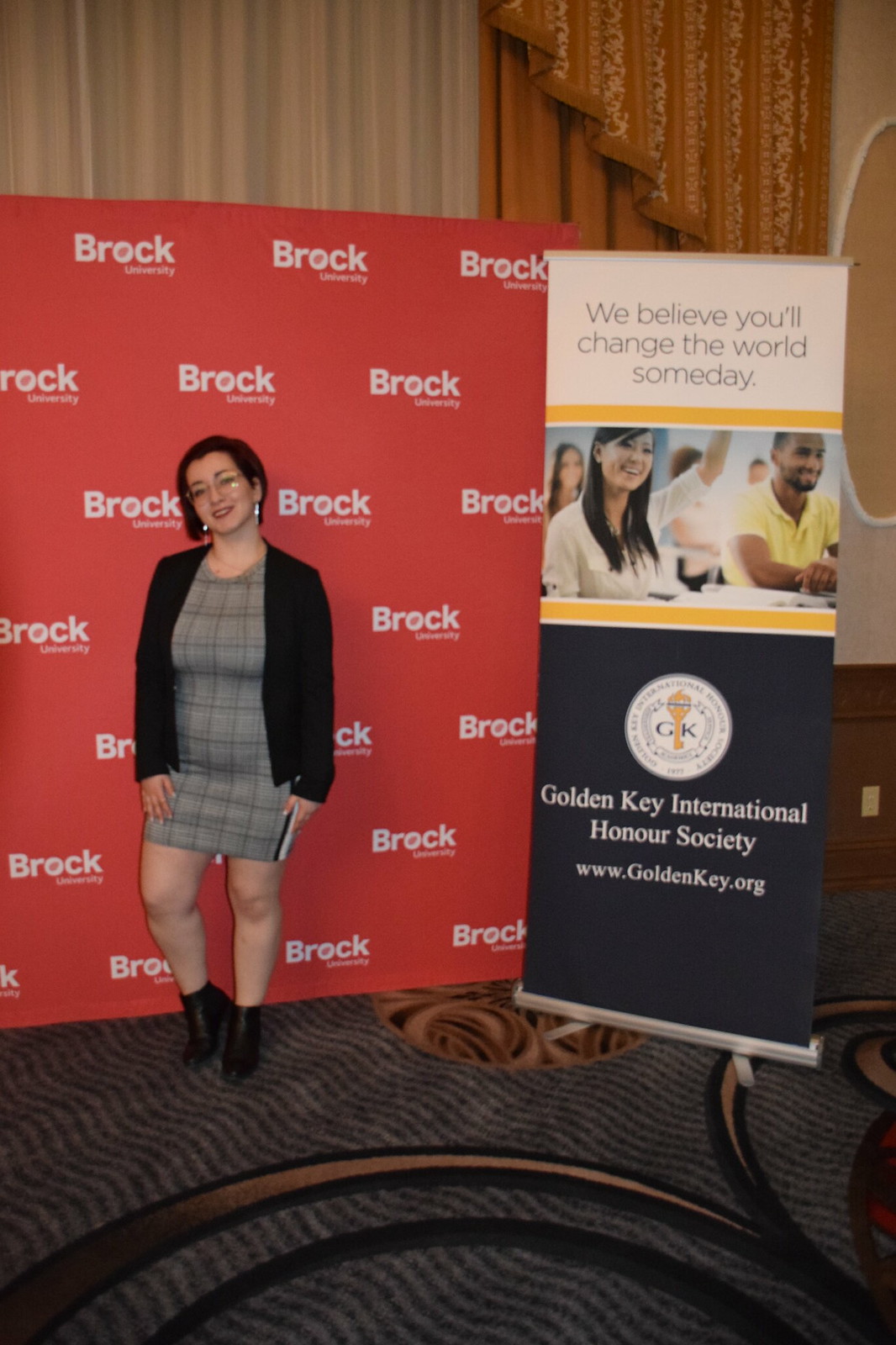In the image, a woman poses confidently for the camera, standing against a prominent red background adorned with repeating Brock University logos in white sans-serif font. She is dressed stylishly in a gray plaid mini dress, layered with an open black sweater. Her ensemble is completed with ankle-length black boots and accessorized with white earrings and eyeglasses. In her hand, she holds an object, which appears to be either a purse or a smartphone. 

Adjacent to her, on the right side, is a banner for the Golden Key International Honor Society. This banner features a detailed design: the upper portion has a white background with black text stating "We believe you'll change the world someday," alongside images of students in a classroom. The lower part of the banner has a dark blue background, a circular logo of the society, and the website www.goldenkey.org displayed in a serif style font.

Further back, the setting includes tan and orange curtains with a distinctive design, all standing on a gray carpet patterned with black and tan circles. The combination of elements adds depth and context to the scene, emphasizing the academic and inspirational environment of Brock University.